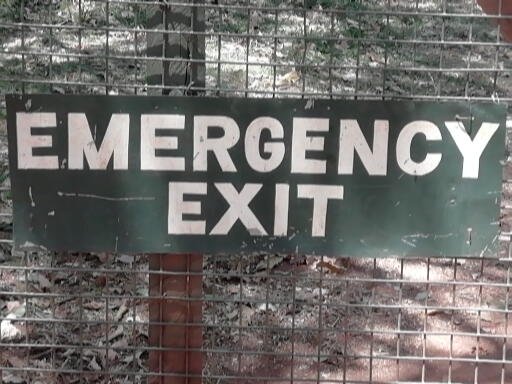The image, captured outdoors, features a dark green metal sign affixed to a see-through metal fence. The sign, which bears the words "EMERGENCY EXIT" in bold white capital letters, displays evident scratches on its surface. Beyond the fence, a wooden pole stands amidst a landscape with patches of green grass interspersed with burned-out areas where bare dirt is visible. The ground is scattered with fallen leaves and small wood chippings. Despite the gray appearance from what seems to be remnants of ashes and dust, the scene is bathed in sunlight, hinting at a bright and sunny day with light streaming through a forested backdrop.